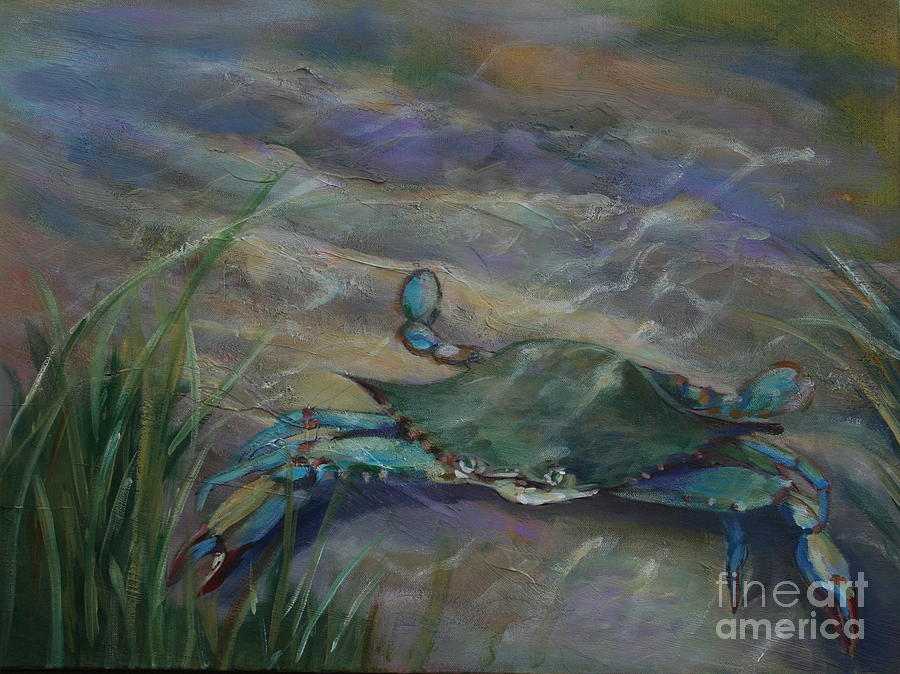In this intricate painting of an underwater scene, the viewer is transported to the seafloor where detailed elements contribute to a rich visual story. In the bottom left corner, green seagrass of varying shades sways gently, captured in fluid, sweeping brushstrokes. More seagrass extends towards the right side of the painting, adding to the sense of depth and movement within the composition.

Central to the scene is a determined crab, painted in dark green and blue hues with striking red detailing on its blue legs. The crab, depicted with white, expressive eyes, appears to be on a mission, reaching out and snipping at the seagrass with its claws. Ripples in the water and the interplay of light create a shimmering effect, illustrating sunlight penetrating through the ocean water and casting dynamic shadows on the sandy seafloor. 

The sandy bottom transitions from a gentle tan to a deep purple, emphasizing the rocks and further enhancing the depth and realism of the scene. The addition of text in the bottom right corner reads "Fine Art America," not detracting but subtly complementing the overall beauty and detail of this underwater tableau.